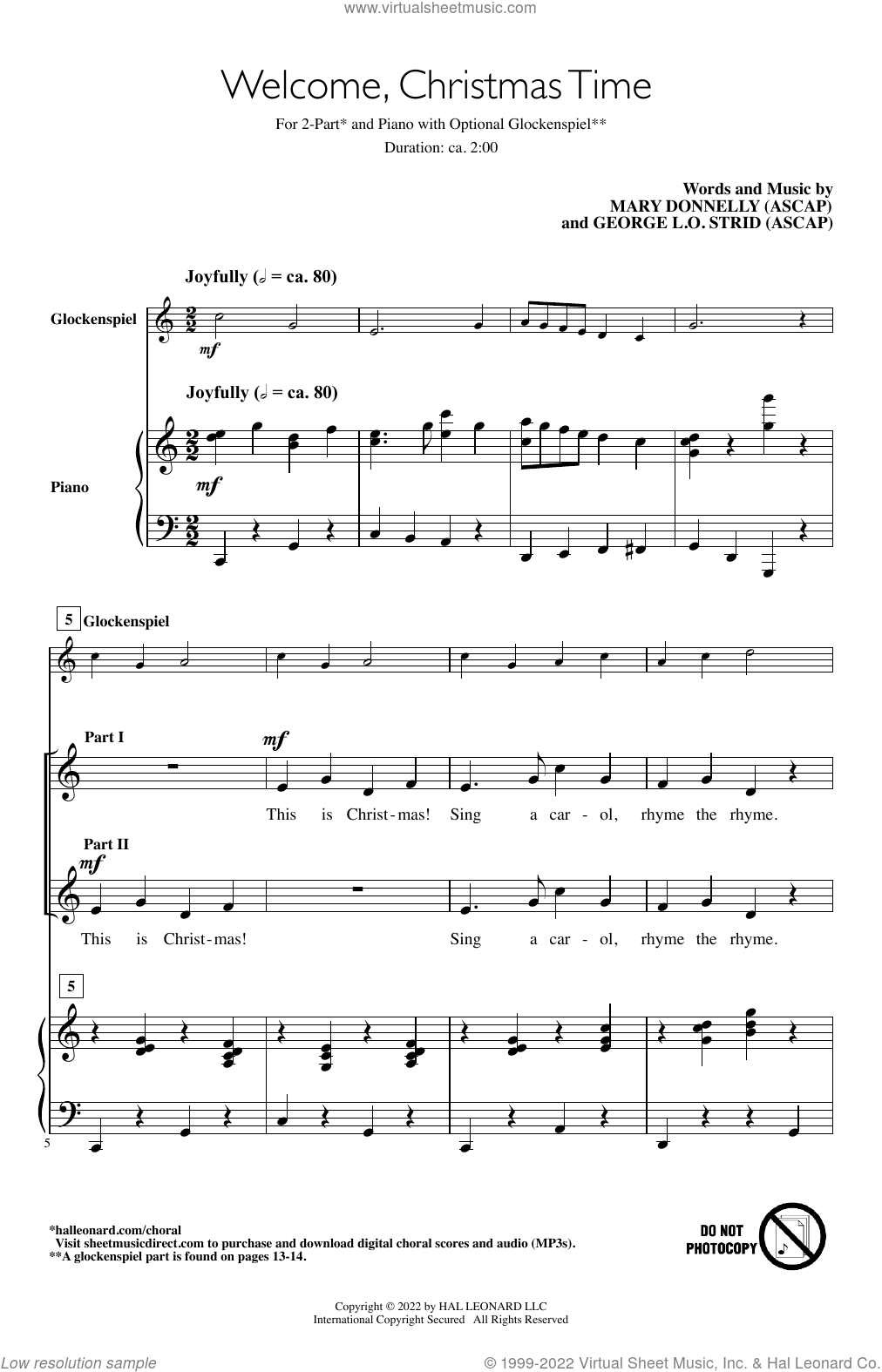This image depicts the sheet music for the Christmas song "Welcome Christmas Time," designed to be played joyfully. At the top of the sheet, the website "www.virtualauthenticmusic.com" is written in black text. Below the website, the song title "Welcome Christmas Time" is prominently displayed in a serif style font, likely Times New Roman, indicating it is a two-part arrangement with a duration of two minutes. The composers, Marty Donnelly (ASCAP) and George L. Strid, are credited beneath the title.

The sheet music is organized into various components, with some sections showing narrower staves than others. It contains a mix of musical notes and lyrics, scattered across a total of eight lines, with the first three lines being narrower than the remaining five. The instructions "joyfully" indicate the intended mood for the performance, and piano parts are included.

At the bottom right corner, a bold warning in black letters states "DO NOT PHOTOCOPY," accompanied by a black circle symbol with an "X" through it, emphasizing the copyright notice.